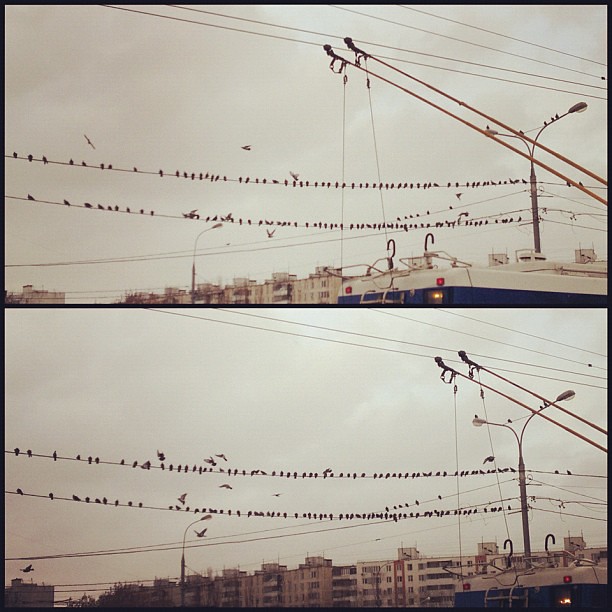The image consists of two nearly identical photographs, one above the other, depicting a cloudy, gray sky backdrop. Both photos capture a bustling urban scene with numerous apartment complexes in the background. A white and blue bus or RV is slightly repositioned between the two images, indicating a slight difference in time or perspective, reminiscent of a picture book style where multiple shots are taken in quick succession.

Cranes with lines reaching to the ground dominate the mid-ground, while the foreground is cluttered with power and telephone lines. These lines are densely populated with small, dark-colored birds, some of which are captured mid-flight. To the far right of the frame, there's a light pole that also hosts a few perched birds. The intricate mesh of wires and the flock of birds create a dynamic contrast against the static background of buildings and the subtle details in the moving bus or RV.